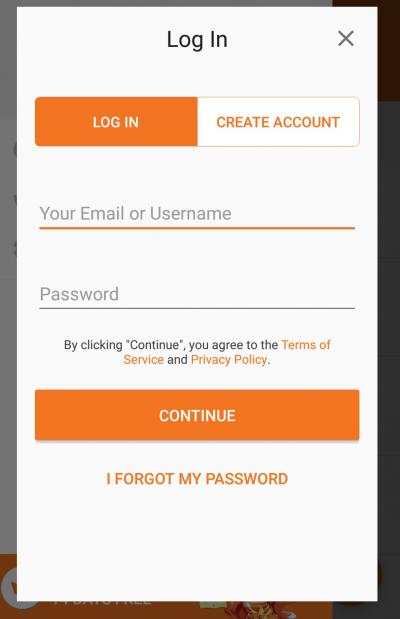The image depicts a login pop-up interface with a predominantly white background. At the top center, the heading "Log In" is displayed in bold black text, accompanied by a gray "X" mark to the right for closing the pop-up. Below the heading, there are two buttons: the left button is colored orange with the text "Log In" in white, while the right button shows "Create Account" with an orange text on a white background.

Beneath these buttons, the central portion of the image features an input field labeled "Your email or username," marked by an orange horizontal line underneath. Following this, there's another input field for the password, indicated by the word "Password" in light gray text and a thin black underline.

Further down, there is a disclaimer stating, "By clicking continue you agree to the Terms of Service and Privacy Policy," with "Terms of Service" and "Privacy Policy" highlighted in orange text. At the bottom of the pop-up, there's a prominent "Continue" button in white text on an orange background. Lastly, beneath this button, the phrase "I forgot my password" appears in orange text.

Overall, the design uses a combination of orange, white, gray, and black colors to create a clear and user-friendly login interface.